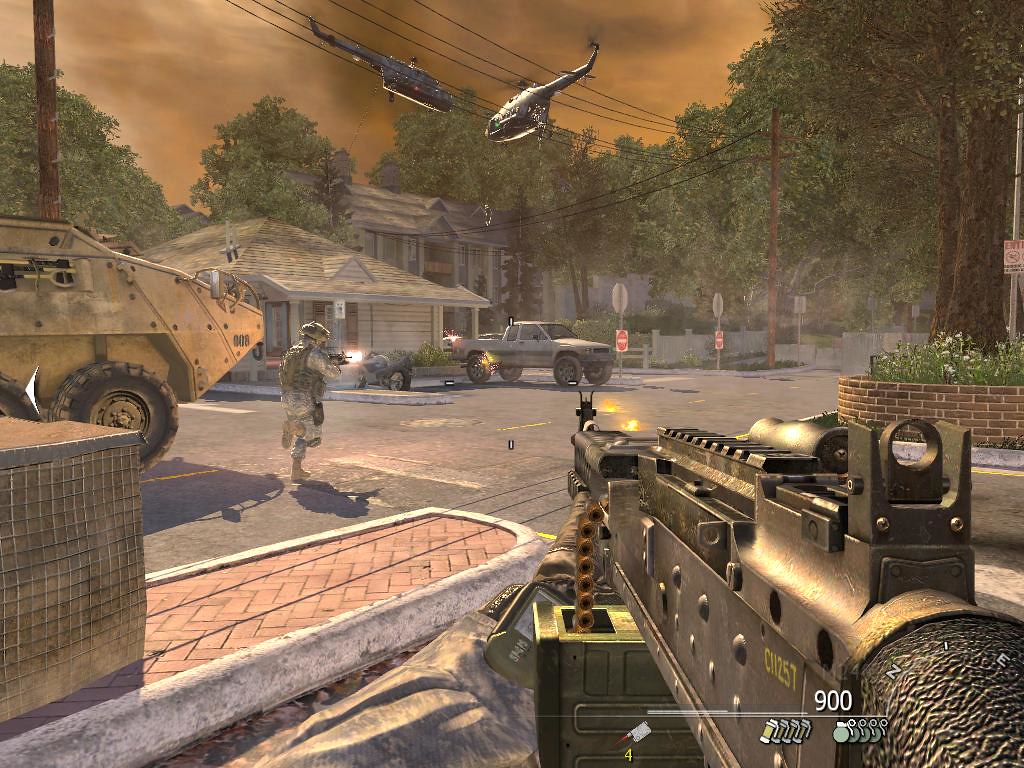This detailed screen capture from a modern first-person shooter video game presents an intense military scenario. The view is from the perspective of a soldier holding a large, camouflaged automatic gun, marked with 'C-11257', with a sight and substantial ammunition visible. The scene unfolds on a residential street featuring a white pickup truck parked in front of a pointed-roof white building. To the left, another armed soldier, donned in camouflage gear and a green helmet, is seen running towards the truck, actively firing a gun with an orange muzzle flash. The environment is teeming with military vehicles, including a Humvee-type yellow vehicle and a beige military tank. Hovering above, two helicopters dominate the reddish-orange, smoky sky, amidst overhead power lines. The backdrop includes numerous green trees, a brick wall with flowers, and intersecting side streets marked with stop signs. The setting is a combat-heavy residential area, complete with telephone poles and a dramatic atmosphere of warfare.